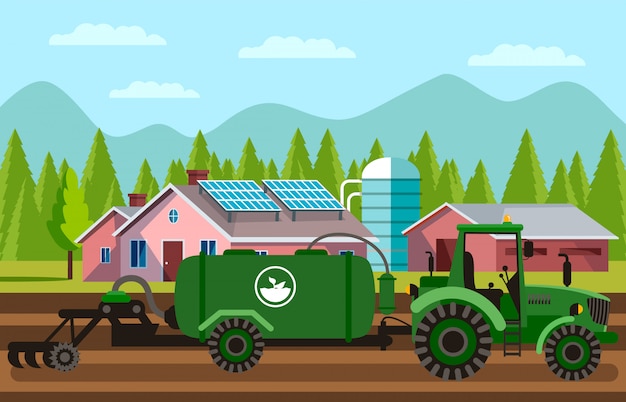This digital print portrays a charming, cartoon-like farm scene, characterized by crisp, clean lines and uniform colors. Set against a sunny blue sky adorned with light white clouds, a jagged mountain range stretches across the background. In front of these mountains, a dense line of triangular evergreen trees in various shades of green rises from different heights, adding to the depth of the image.

In the mid-ground, a vibrant pink farmhouse with solar panels on its roof stands out. This house has a burgundy door and is complemented by a barn of a darker shade of pink, adjacent to a blue silo. The farmhouse and barn form a picturesque rural setting that spans a significant portion of the image.

Dominating the foreground is a large green tractor, stationary on a dirt path. It is attached to a green tank with illustrations suggesting either a watering or pesticide system, complete with hoses and digging claws designed to till the soil. The tractor and its equipment imply active farm work, preparing the land for planting seeds.

Overall, the scene is a harmonious blend of natural and agricultural elements, vividly capturing the essence of a serene and productive farm on a clear, sunny day.